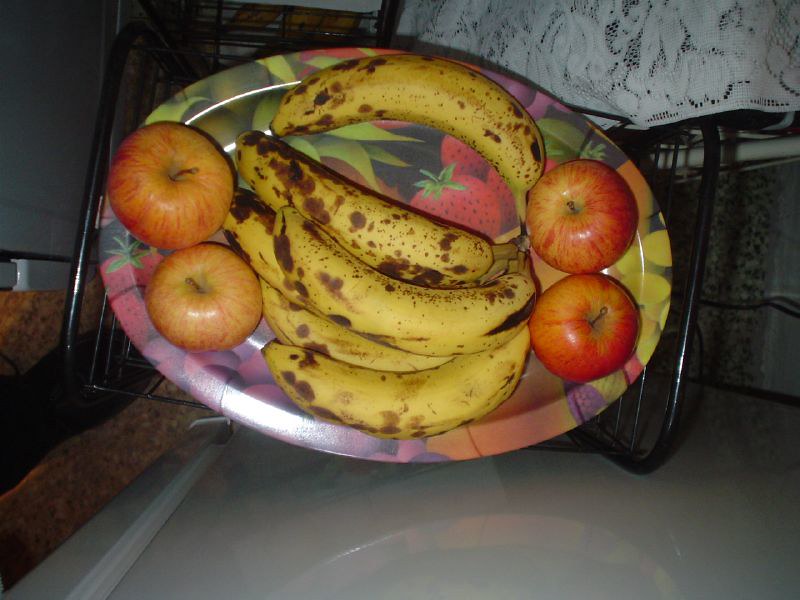In the close-up image, we see an oval-shaped tree serving tray placed within a black metal basket-like container. The tray is filled with an assortment of fruits, meticulously arranged for a visually appealing display. The fruits include two reddish-golden apples on the left, six very ripe bananas in the center, characterized by their bright yellow skin adorned with dark brown marks and spots, indicating their ripeness. On the right side of the bananas, there are two additional reddish-golden apples, mirroring the arrangement on the left. The contrast between the vibrant colors of the apples and the well-ripened bananas creates a harmonious and appetizing presentation.